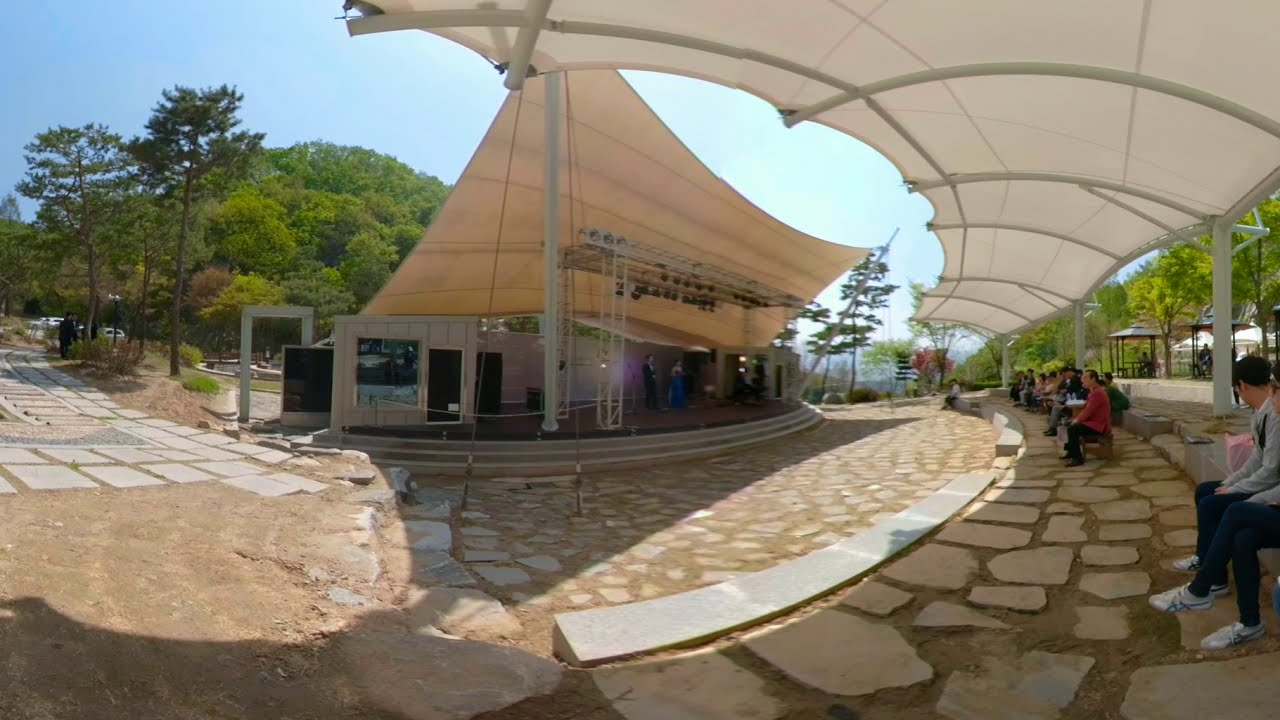The image captures an outdoor performance area featuring a rounded stage with cement steps and a large white canvas tarp suspended by steel girders, providing shade for the performers and audience. The foreground showcases a flat, stone-paved floor composed of variously shaped white stones with dirt acting as mortar. To the right, there's a seating area with three to four rows of cement slabs for the audience, also covered by a white canvas held up by curved steel poles. People sit wearing long sleeves and pants, suggesting a cool day, and they are focused on two performers on the stage. Surrounding the area are trees, making it appear like a public museum or a tourist spot, possibly with shuttle services, as suggested by the stone walkways and informational panels under additional canvas overhangs. The blue sky adds to the serene and leisurely atmosphere of the scene.